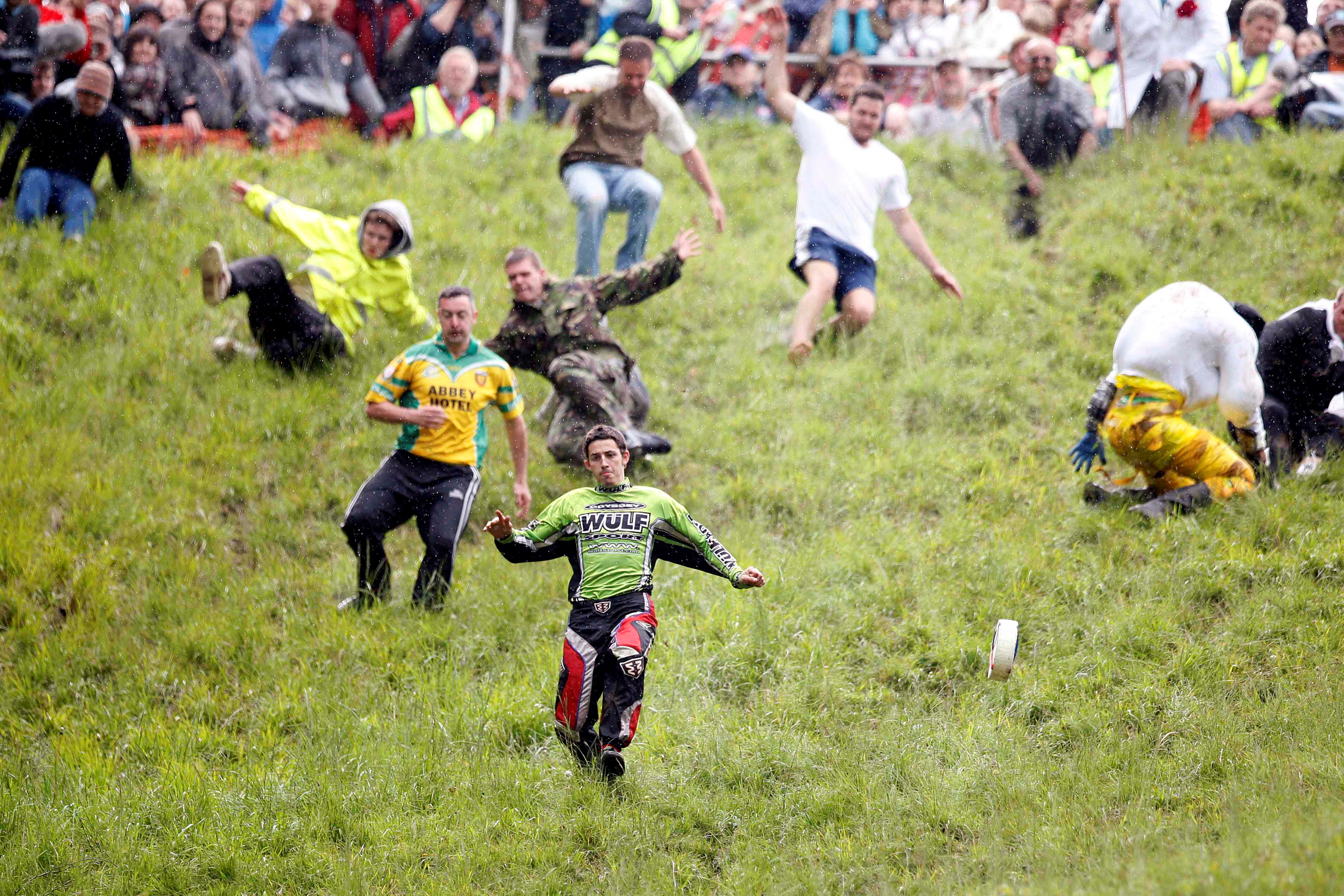In the foreground, a group of predominantly men are energetically running and tumbling down a steep grassy hill. Most of the hill, taking up about four-fifths of the image, is vibrant green. The central figure is clad in a green long-sleeved shirt with "W.U.L.F" printed on it, paired with black and red pants. Behind him, a man wears a yellow and blue-green shirt with unreadable text and black pants featuring white stripes. There's also a man in what seems to be army fatigues and another in a light green jacket with black pants, who appears to be losing his balance.

A little further up, another man can be seen, donning a white and brown shirt combined with blue jeans. On the far right, is an unusual figure in yellow pants who looks AI-generated. Nearby, a small white disc is rolling down the hill, possibly the object these individuals are chasing. To the left of the army-clad man, a figure wearing a white t-shirt and blue shorts with white stripes seems to be in the midst of sliding down the slope. 

In the far background, a large crowd of spectators watches intently from behind a gated fence. The top fifth of the image is densely packed with these onlookers, creating a sense of a lively and chaotic scene perhaps at some type of event involving a race or competition.